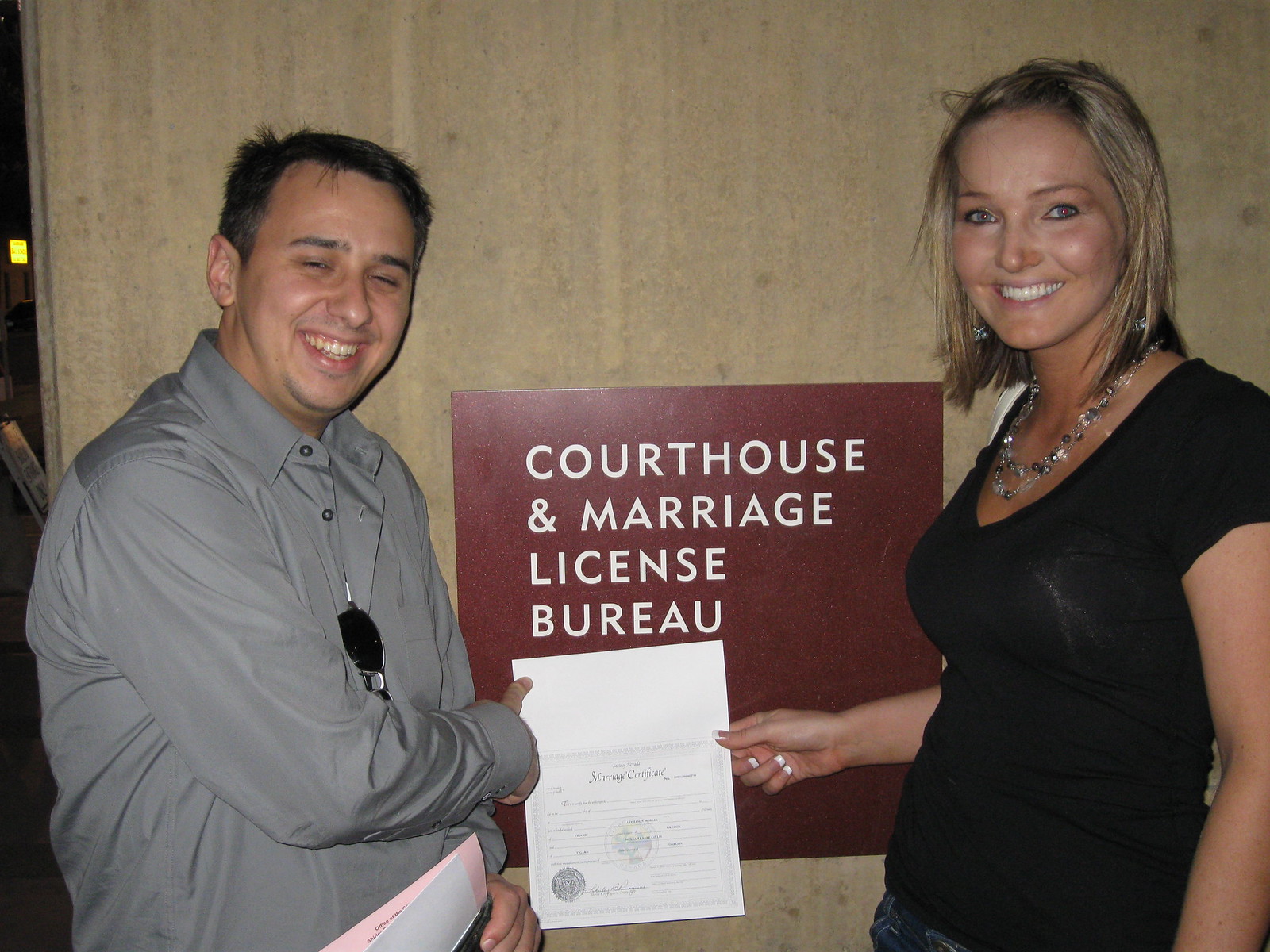This photograph captures a joyous moment of a newly married couple outside the Courthouse and Marriage License Bureau. On the left stands a man with short black hair and a clean-shaven face, wearing a long-sleeved gray button-up shirt. He is beaming broadly, his eyes shut in delight, and through his shirt, a pair of glasses can be seen tucked in. In his other hand, he holds a pink and white paper. On his right is a woman with blonde hair and blue eyes, dressed in a short-sleeved black top. She wears a distinct bangle necklace and has her nails painted white. Both of them are holding up what appears to be their marriage certificate with their right hands, proudly displaying it underneath a sign that reads "Courthouse and Marriage License Bureau" on a rust-colored, wood-textured wall. Their expressions and the setting clearly convey the happiness of their special day.